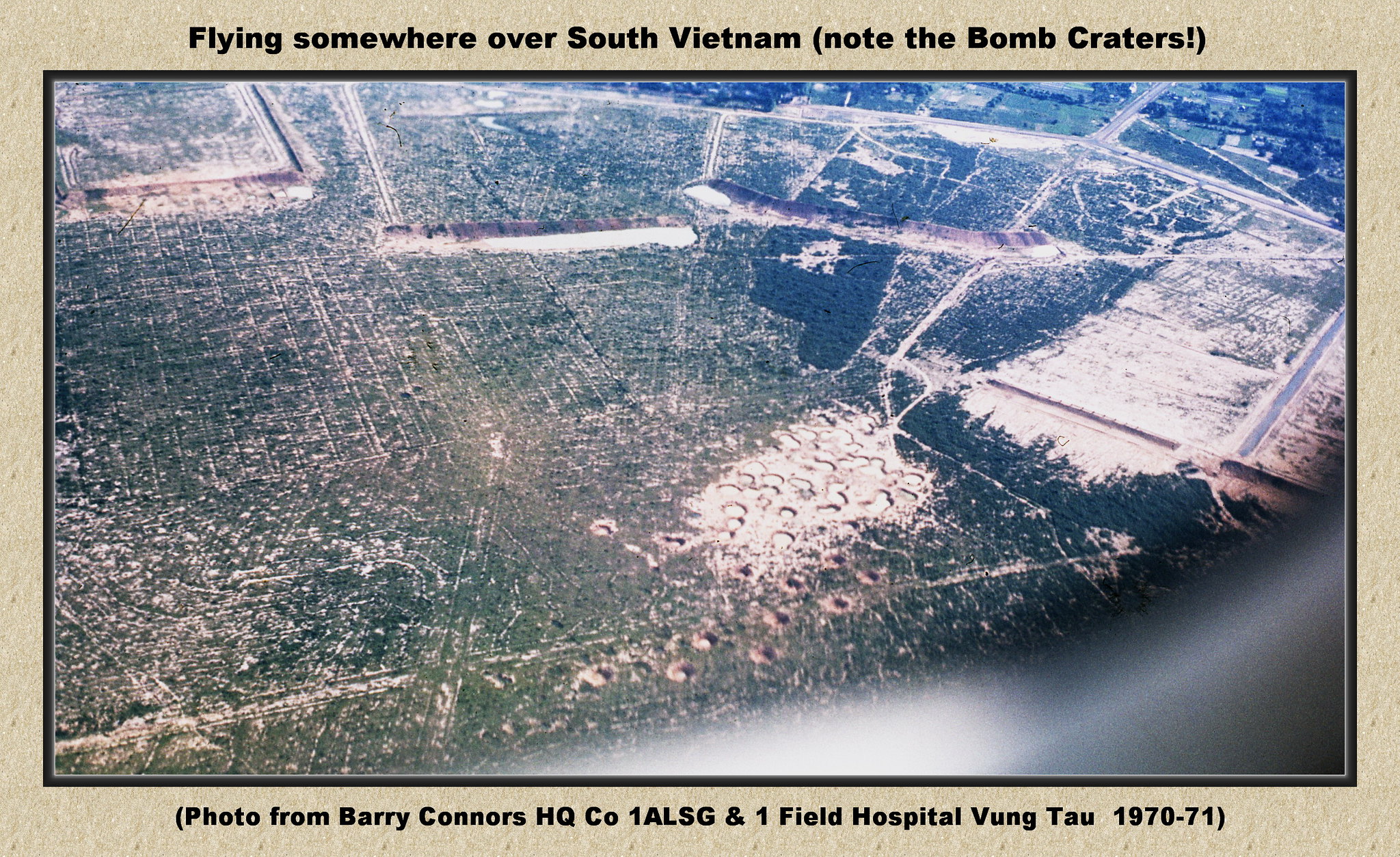This image, a rectangular, horizontal color photograph framed by a light gray, sand-textured border, shows an aerial view of South Vietnam. The photo is encapsulated by black ink text on the top border stating, "flying somewhere over South Vietnam (note the bomb craters)." The image showcases a vivid landscape where the left side predominantly features green farmlands divided into plots, while the right side displays trees and a sandy area. In the photograph's lower right corner, there are numerous white craters, indicating bomb damage, with what appear to be untouched neighborhoods in the upper right. Below the photograph, another caption in the beige border reads, "(photo from Barry Conner's HQCO-1ALSG and One Field Hospital, Vung Tau, 1970-71)." The detailed topography includes a mix of brown and white regions, possibly representing additional buildings and undamaged areas amidst the war-affected landscape.